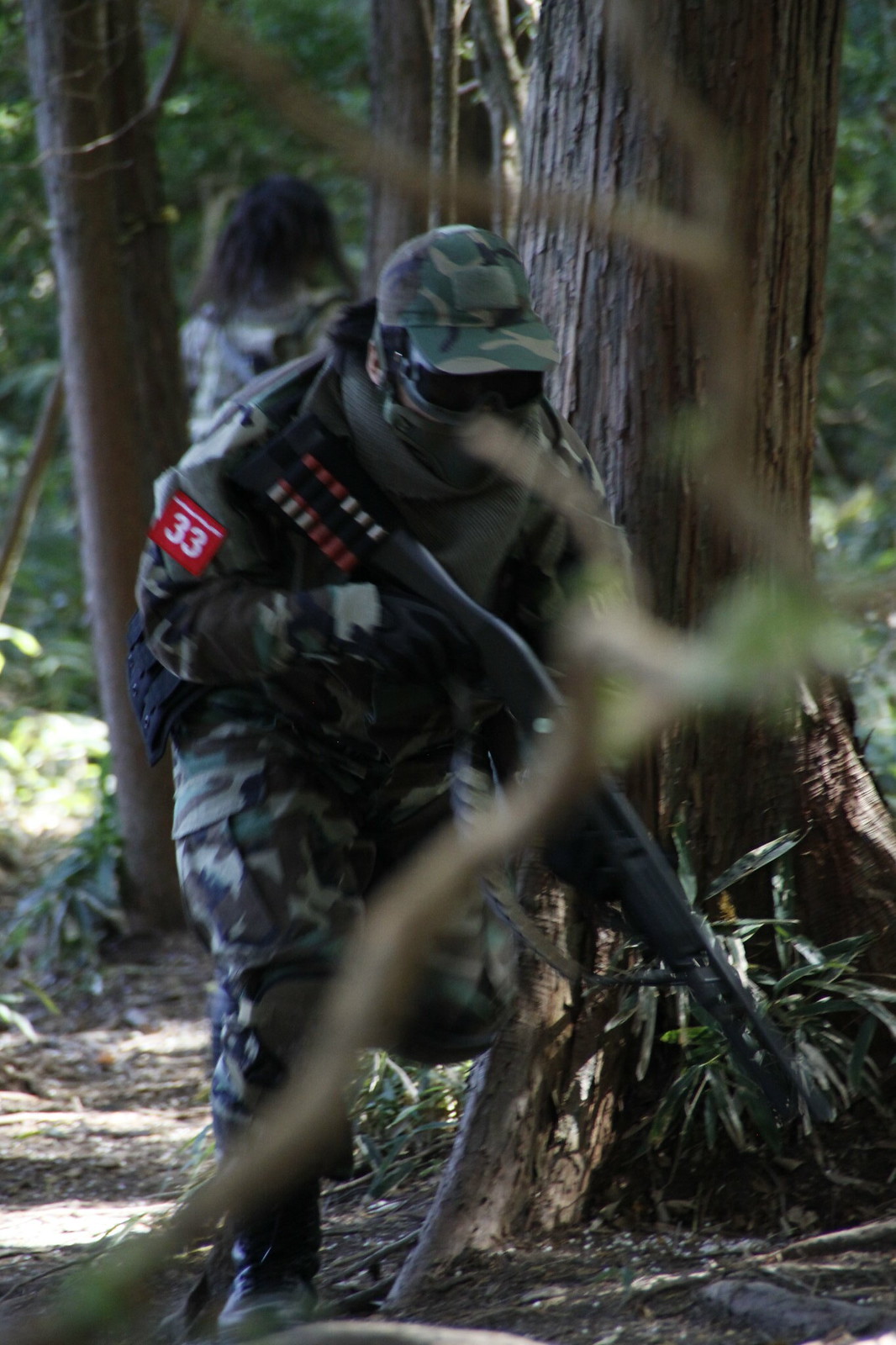In this detailed photo, a soldier is captured in a dynamic, running position amidst a dense forest. Dressed in full camouflage, including a hat, mask, sunglasses, and knee pads, he is clearly geared up for a tactical mission. The uniform features a prominent red patch with white letters that read "33," likely identifying him for a game or exercise. The soldier wields a long, black shotgun with six red shells strapped to its stock. He is positioned near a large tree, partially crouched as if moving towards a target or taking cover. Just behind him, another figure, partially visible, appears to be a teammate, turned away and looking in the opposite direction. The lush foliage and trees of the forest set a vivid natural backdrop, enhancing the sense of action and urgency in the scene.